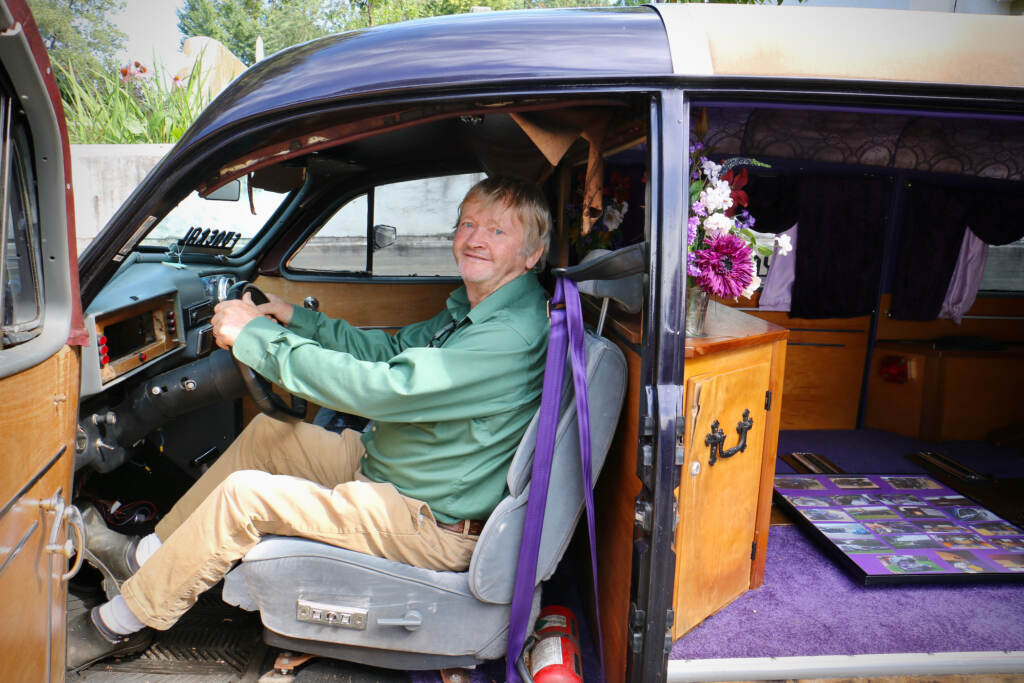An older person is seated in the driver's seat of a van with the driver's side door open. This person, identifiable by flecks of gray in their hair and subtle wrinkles, is wearing a teal-colored, long-sleeved shirt with a collar, brown pants, white socks, and brown shoes. Their hands are on the steering wheel, and although they are not wearing it, the seatbelt appears to be purple. The seat they are sitting in is gray, and the dashboard is also gray. The top of the van is black while the rear interior is tan. The back area of the van features a purple carpet, wooden furniture including cabinets, and possibly a TV. There are also picture frames on the floor and flowers on one of the cabinets.